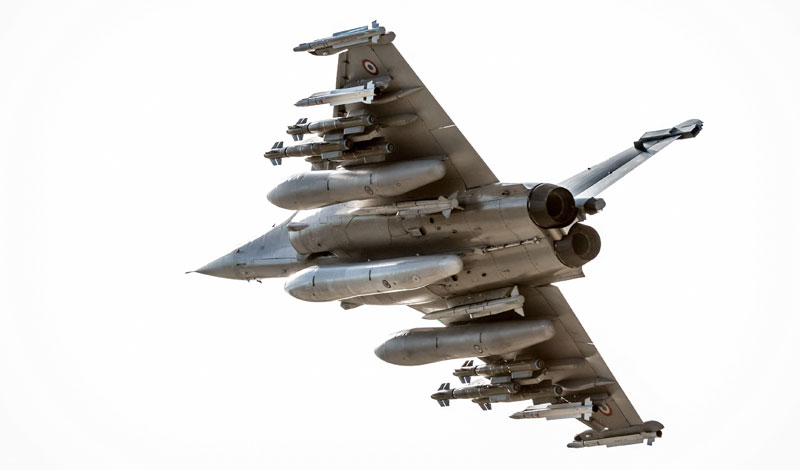The image depicts a highly detailed, color photograph of a silver, triangular-shaped fighter jet viewed from below against a white background. The sleek, gray jet is equipped with an array of military attachments, including white and gray missiles, some with wings, and several large, cylindrical rockets prominently mounted beneath its wings. The jet features a needle-point nose and two powerful rocket exhausts at the rear. The scene captures the plane in mid-air, highlighted by the bright and natural lighting which adds to the clarity and sharpness of the image. The stark white sky in the background further emphasizes the jet's formidable design and armament, giving a clear and unobstructed view of the aircraft.